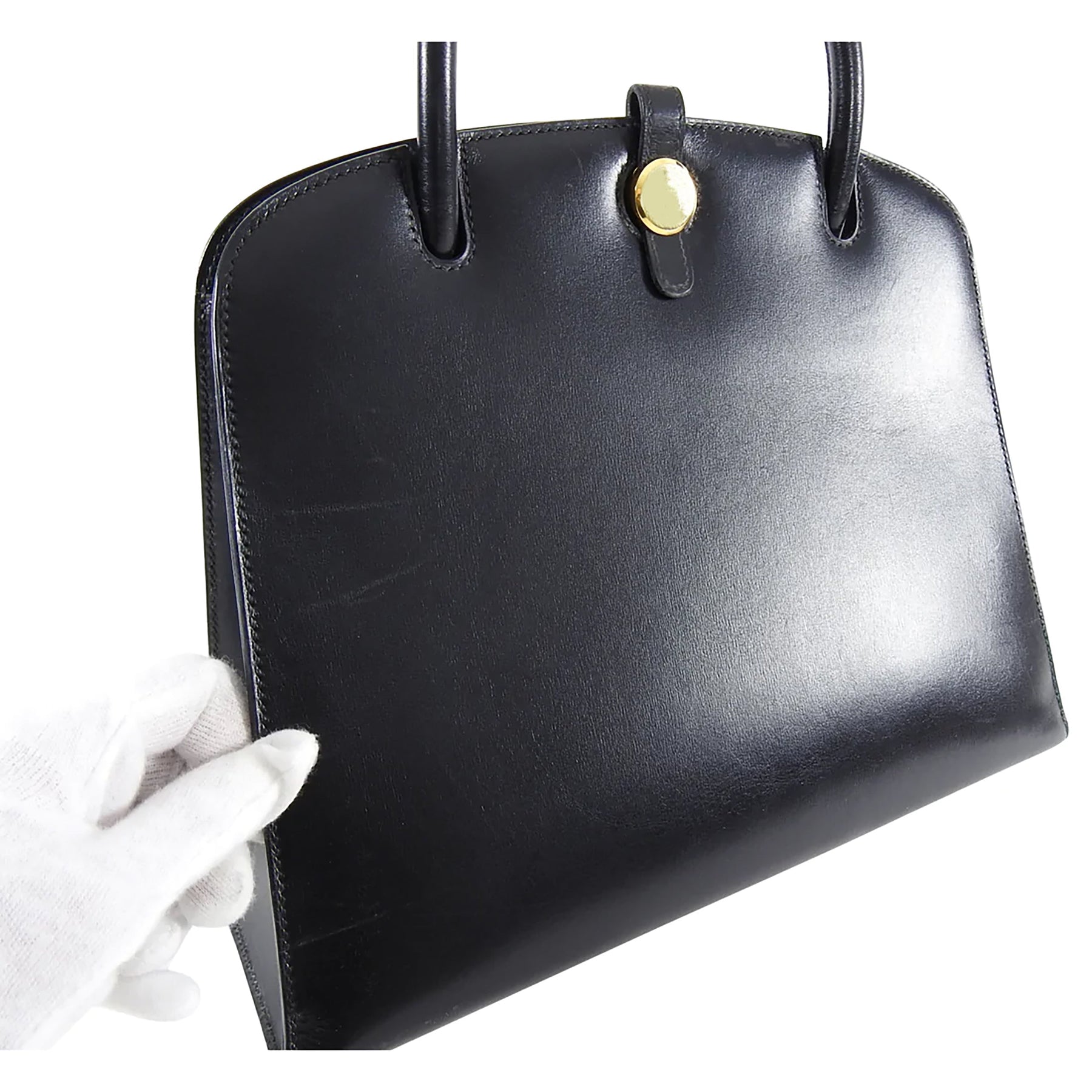In this very close-up, black and white photograph, a gloved hand is seen holding a small, plain black purse. The purse, which appears to be made of shiny black leather, features a single strap and a round, gold button closure in the center, which serves as a latch to seal the top. The image has been edited to remove the background, drawing all attention to the purse and the white-gloved hand that holds it. The purse, approximately 12 inches across, has a sleek and polished finish with a couple of visible scratches on the left side and some white reflections highlighting its glossy texture. The overall design is minimalistic, with no additional patterns, images, or writing adorning the surface.